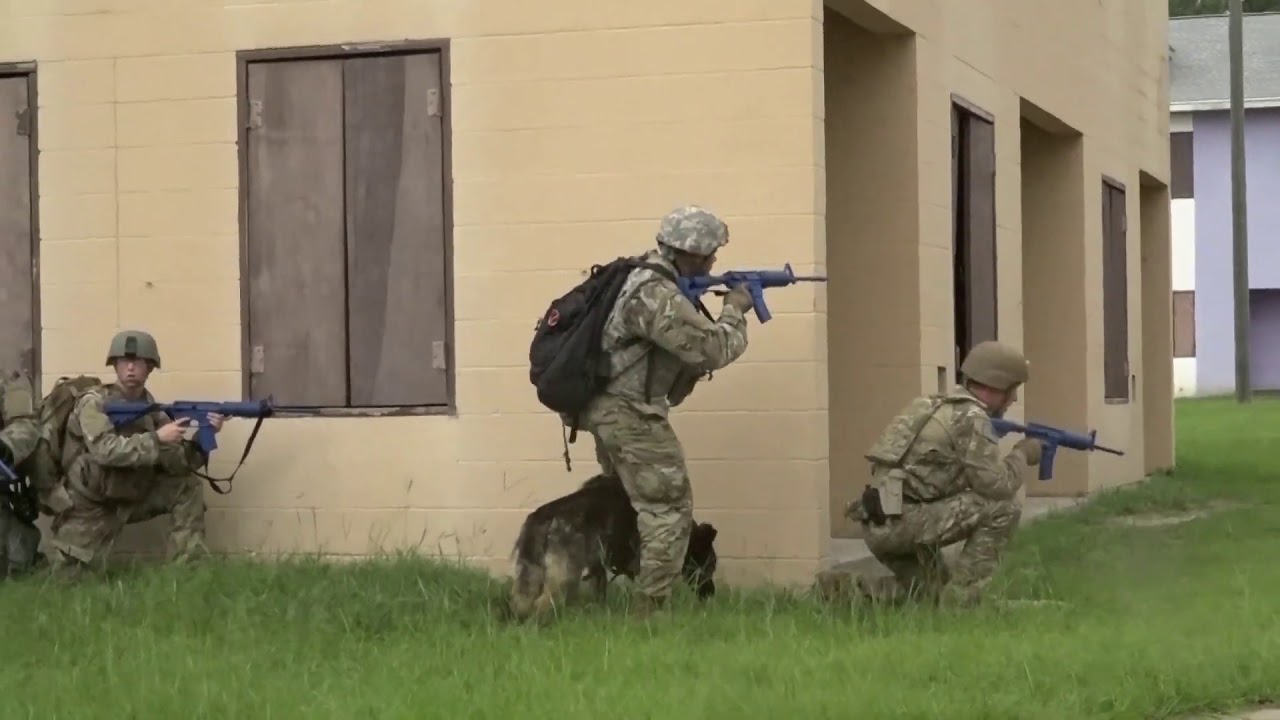The image depicts a military training scene centered around a tan, white, and gray cinder block building with closed wooden shutters. Positioned among slightly tall, light green grass, three soldiers in light green and tan camouflage and helmets are seen. The middle soldier stands at the building's corner with a blue automatic rifle and a dog, likely a German Shepherd, between his legs. One soldier crouches to his right and another crouches to his left. Each soldier carries a similarly camouflaged backpack, except for one sporting a black backpack. They all appear to be scoping out the area, with their focus directed towards an unseen point, possibly a second white building in the background, suggesting a diligent examination of their surroundings.